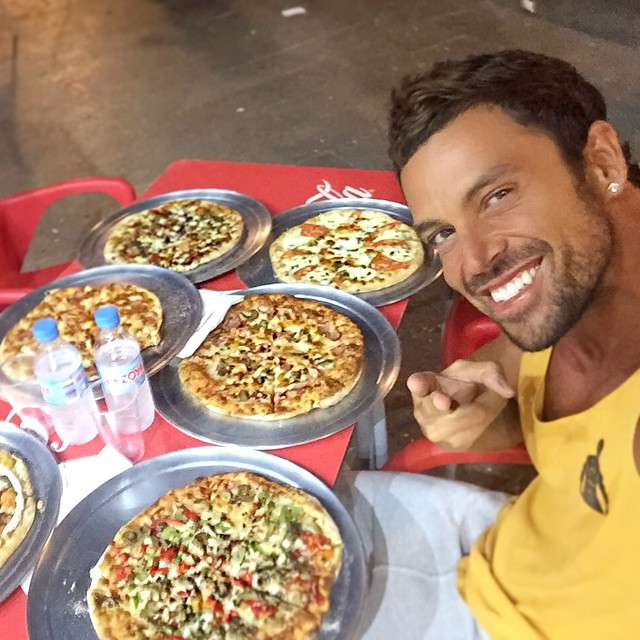The image features a young man, possibly around 25 years old, with short dark hair and a light stubble, sitting at a red tablecloth-covered table, possibly branded with the Coca-Cola logo. He's seated in a red chair with an empty red chair beside him. He wears a yellow tank top with a silhouette emblem on the chest and grayish-white pants. His left ear has a small diamond stud, and he is smiling brightly, showing his white teeth, while pointing a peace sign with his right hand towards the camera as he takes a selfie. The table is set with six pizzas on silver platters, all with different toppings and untouched, along with two water bottles with blue caps and two empty plastic cups. The background is a gray, concrete floor.